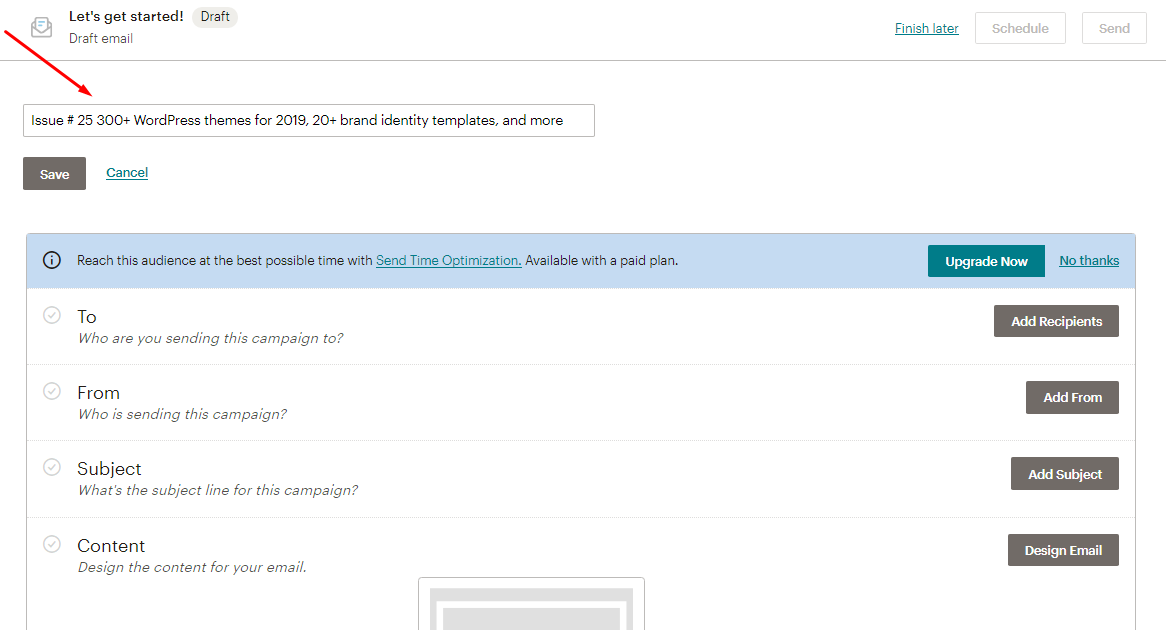A clean and detailed caption for the described image might be:

"This is a screenshot of an email composition interface. In the upper left corner, text reads 'Let's Get Started,' with 'Draft Email' below it and a mail inbox icon to the left. To the right of 'Let's Get Started,' the word 'Draft' is displayed. In the upper right corner, options to 'Finish Later,' 'Schedule,' and 'Send' are available, with 'Schedule' and 'Send' being clickable buttons.

Prominently displayed in the center is a large rectangle highlighting the text: 'Issue Number 25, 300+ WordPress Themes for $219, 20+ Brand Identity Templates and More,' with a red arrow pointing to it from the upper left. Below this section, there are options to 'Save' with a button and 'Cancel' with a link.

Further down, a blue bar advises, 'Reach this audience at the best possible time with Send Time Optimization available with a paid plan,' offering buttons to 'Upgrade Now' or say 'No Thanks.' Underneath this, four different email entries are visible, showing details of the recipients, senders, subject lines, and email content."